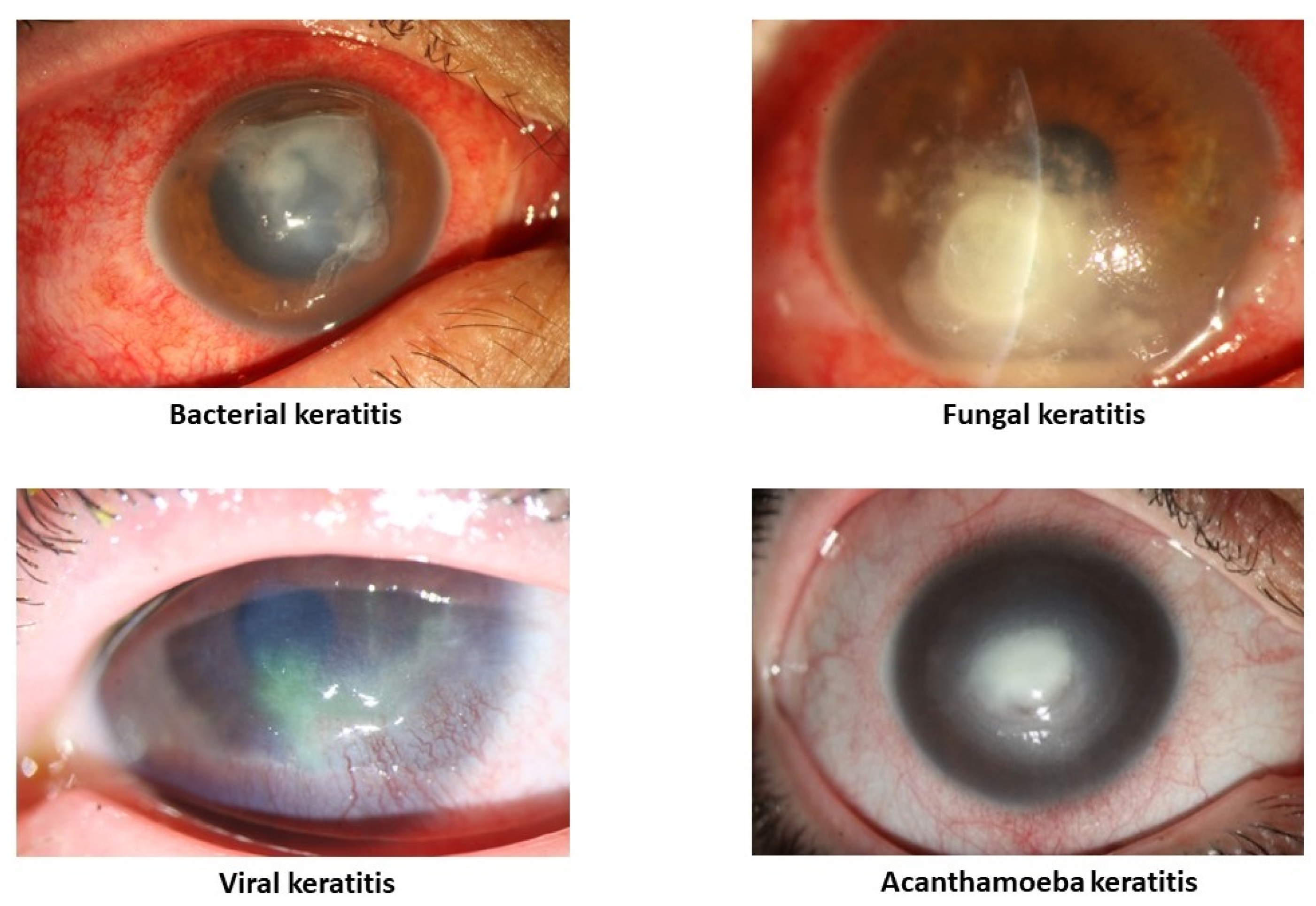This medical diagnostic chart features four up-close photographs of human eyes, each illustrating different types of keratitis, a serious eye condition. The eyes in each image exhibit signs of distress, such as redness and discoloration, indicating an unhealthy state. The images are arranged in a two-by-two grid, with each eye condition labeled in black print, with only the first letter capitalized. 

In the upper left, "Bacterial keratitis" shows an eye with pronounced redness in the sclera, suggesting a severe infection. The upper right image, labeled "Fungal keratitis," displays similar symptoms with red, inflamed veins evident in the eye. On the bottom left, "Viral keratitis" is depicted, marked by noticeable blood vessels that appear inflamed within the white part of the eye. The bottom right image labels "Acanthamoeba keratitis," characterized by red veins and discoloration, signifying an acute eye infection.

Each photograph clearly underlines the severity of these distinct types of keratitis, illuminating the critical need for medical attention and treatment.